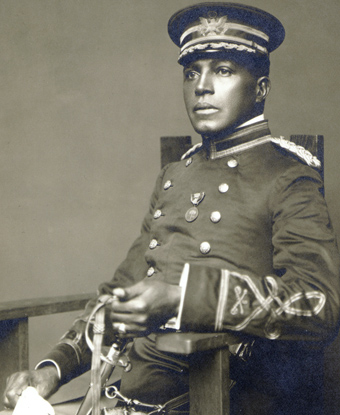In a black and white photograph, a Black man is seated on a wooden chair, his body and gaze angled towards the left. He wears a military uniform, consisting of a long-sleeved gray jacket with white buttons running from his chest to his waist, adorned with medals and golden tassels on the shoulders. On his head, he sports a military cap featuring an eagle emblem. His expression is tense, with fearful eyes and stiff lips, suggesting apprehension about something unseen. His left arm rests on the chair, draped with a silver chain, while his right hand tightly grips a white rag. The photo captures intricate details such as the individual buttons on his jacket and the ribbons and markings on his hat, creating a vivid portrayal of his anxious yet resolute demeanor.